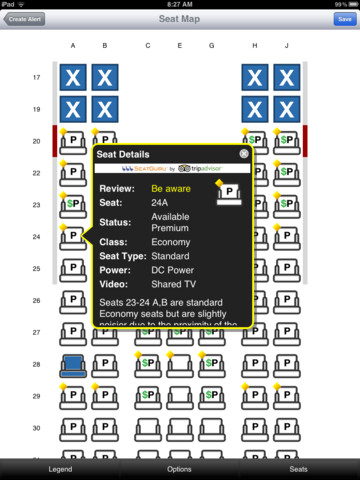The image depicts an Apple iPad displaying a screen with an app interface. The top section of the interface features a navigation bar. On the top left, there is a "Create Alert" button, while on the top right, a "Save" button is highlighted in blue and white. Below this navigation bar, the main content area has a white background with a detailed seat map layout. 

On the seat map, columns are labeled from left to right as A, B, C, E, G, H, and J. Along the left side, row numbers are listed vertically: 17, 19, 20, 22, 23, 24, 25, 26, 27, 28, 29, and 30. Prominently in the center of the screen, there is a black rectangular pop-up window with yellow trim on its edges. The header of this pop-up window reads "Seat Details" on the top left corner.